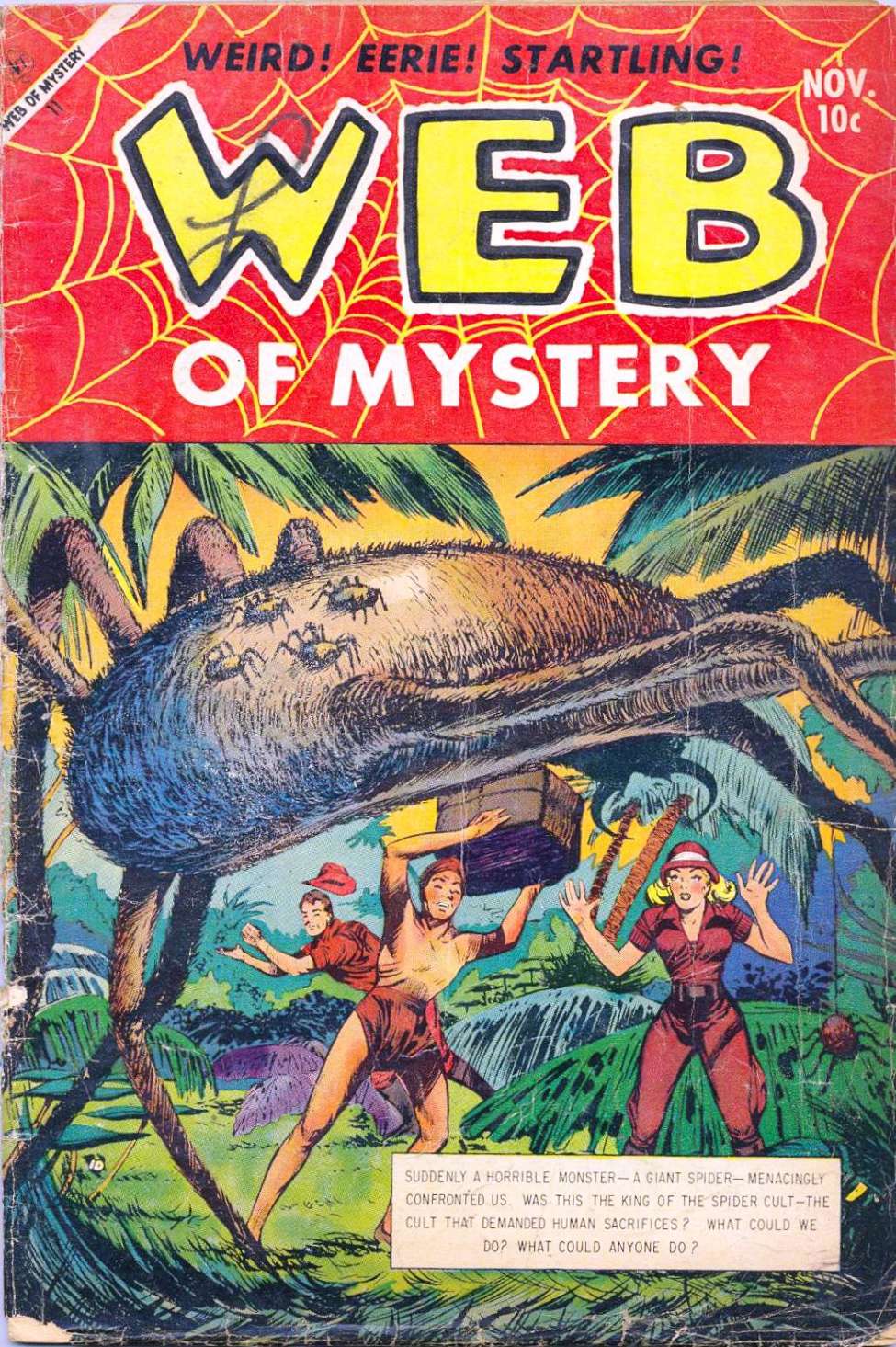The image is a vintage comic book cover, likely from the 1940s or 1950s, titled "Web of Mystery." The top third of the cover features a bold red background with a striking yellow spider web. Prominently across the top, the words "Weird," "Eerie," and "Startling" are displayed in black, with the title "Web of Mystery" written in large yellow letters outlined in black and white.

Centered in the scene is a dramatic tableau: a Tarzan-like figure in a red loincloth is brandishing a box, seemingly poised to strike. He is accompanied by a blonde woman in safari gear who appears terrified, caught in mid-scream with her hands raised. Behind them, advancing menacingly, is a colossal spider, carrying smaller spiders on its back. Another adventurer, also dressed in safari attire, stands behind the duo, contributing to the chaotic sense of danger.

In the top left corner, the cover notes the issue's release as "NOV" and its price at ten cents. Below the central illustration, a tan box with black outlines contains chilling text: "Suddenly a horrible monster, a giant spider menacingly confronted us. Was this the king of the spider cult? The cult that demanded human sacrifices? What could we do? What could anyone do?" The gripping narrative and dynamic imagery encapsulate the thrilling suspense typical of pulp comics from this era.